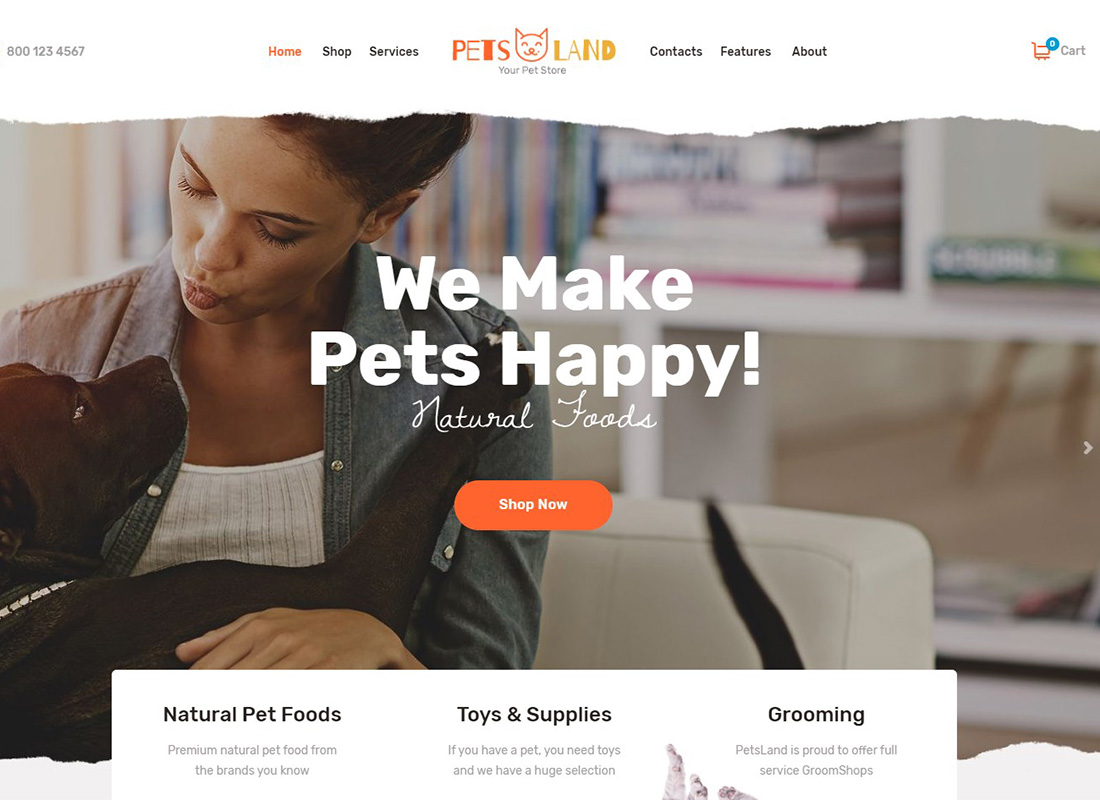The website for Pets Land features vibrant orange and red lettering for the company name, "P-E-T-S," with a slight gradient. Central to the page is a logo of a pet's face, accompanied by the tagline "Your Pet Store" in small print below.

At the top navigation bar, the 'Home' button is prominently displayed in orange, while options for 'Shop,' 'Services,' 'Contacts,' 'Features,' and 'About' are in black. An orange shopping cart icon is positioned to the right, marked with a blue circle indicating the number of items.

The main image showcases an affectionate moment between a girl and her black dog. The girl, dressed in a white shirt with a gray jacket, makes a kissy face at the dog, which gazes up at her while lying in her arms. She is seated on a white leather sofa, with the dog's black tail visible and slightly elevated.

Overlaying this touching scene, bold white text declares, "We make pets happy," with a subscript, "Natural foods," beneath it. An inviting orange circle bearing the words "Shop Now" is also present. 

Further down, the page advertises a selection of natural pet foods, toys, and supplies, alongside grooming services, though the text is partially obscured.